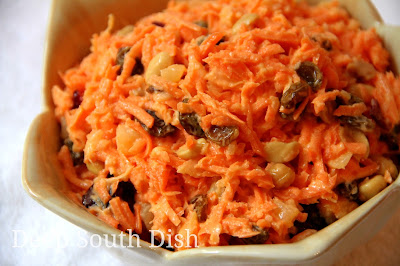This is a high-definition, close-up image of a rice dish presented in a unique, light brown bowl with a jagged, petal-like rim, almost resembling a flower. The rice inside is interspersed with dark orange and black strips, which might be shredded fish, vegetables, or meat. The bowl is placed on a white background, possibly a tissue or paper. At the bottom corner of the image, there is white text partially blending into the white surface, making it hard to read; the legible part mentions "south dish." The detailed composition and presentation suggest it could be a photo taken by a food blogger.